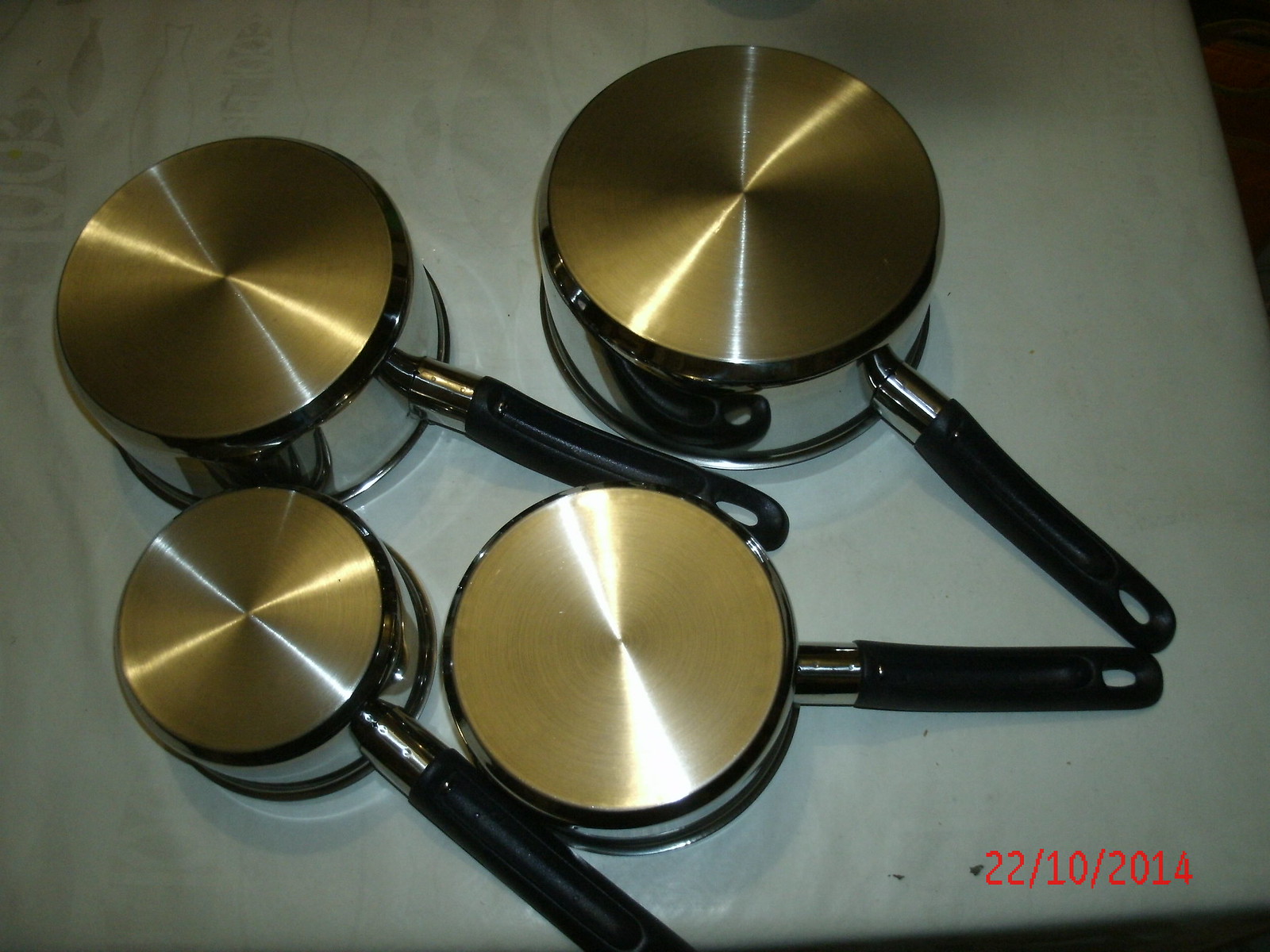This photograph, taken on October 22, 2014, depicts a close-up of four upside-down pots of various sizes, neatly arranged on a white surface that resembles a marble countertop or a white sheet. The pots' bottoms, which are turned towards the viewer, exhibit a highly reflective, criss-crossed light pattern, suggesting a brushed silver finish with a brassy or gold hue. Each pot is equipped with black handles that have loops for hanging, with a small silver section connecting the handle to the pot. The rims of the pots also appear to have a black trim. The smallest pot is positioned in the lower left corner, with progressively larger pots arranged towards the upper left and upper right. The black handles are facing more or less to the right side of the image. There is faint, white lettering in the upper left corner of the surface beneath the pots, hinting at an image or text partially visible through the backdrop. In the bottom right corner of the photograph, the date "22/10/2014" is displayed in red text.